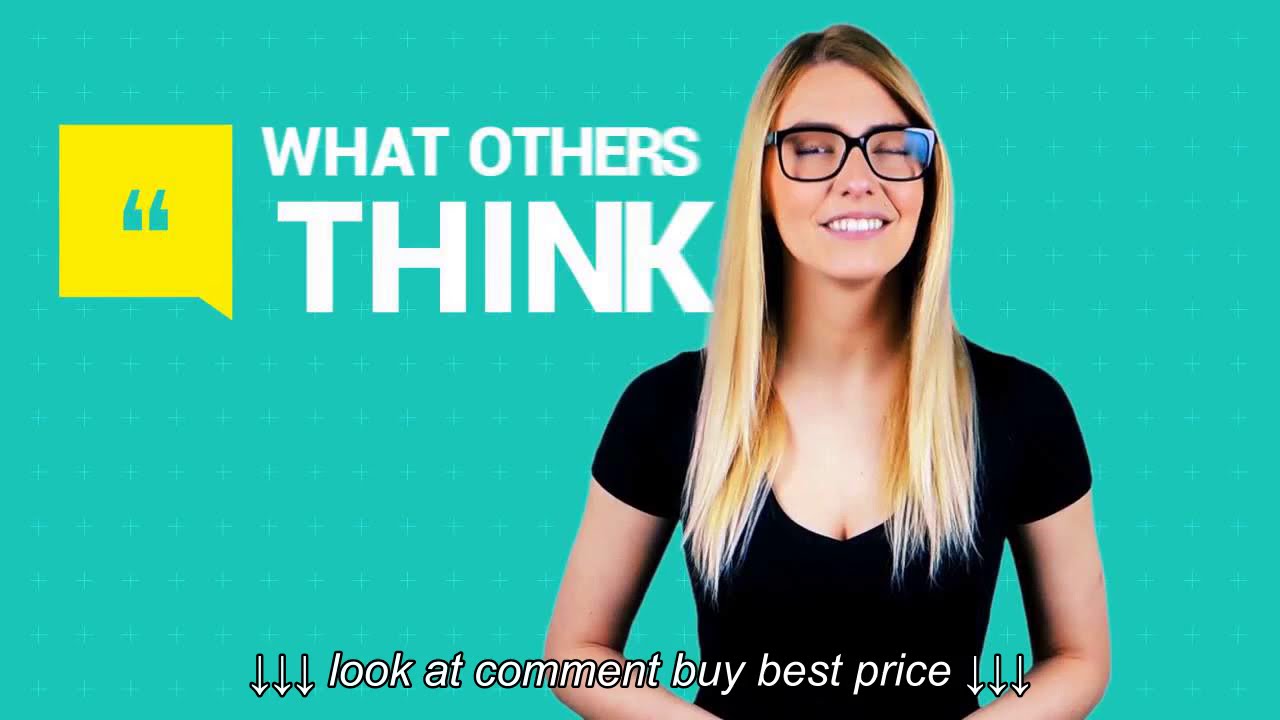This promotional slide features a woman with long blonde hair and dark roots, wearing a black top and large black-rimmed glasses. Her eyes are slightly shut, giving the impression of a mid-blink, yet she has a pleasant smile showcasing her white teeth. The background is a solid aqua or bluish-green color, adorned with a subtle pattern of faint pluses. To the left of her head, in all capital white letters, is the text "WHAT OTHERS THINK," with the word "THINK" emphasized in bold. Left of this text is a large yellow square containing a green quotation mark. At the bottom of the image, a directive reads "LOOK AT COMMENT, BUY BEST PRICE," flanked by three downward-pointing arrows on each side.